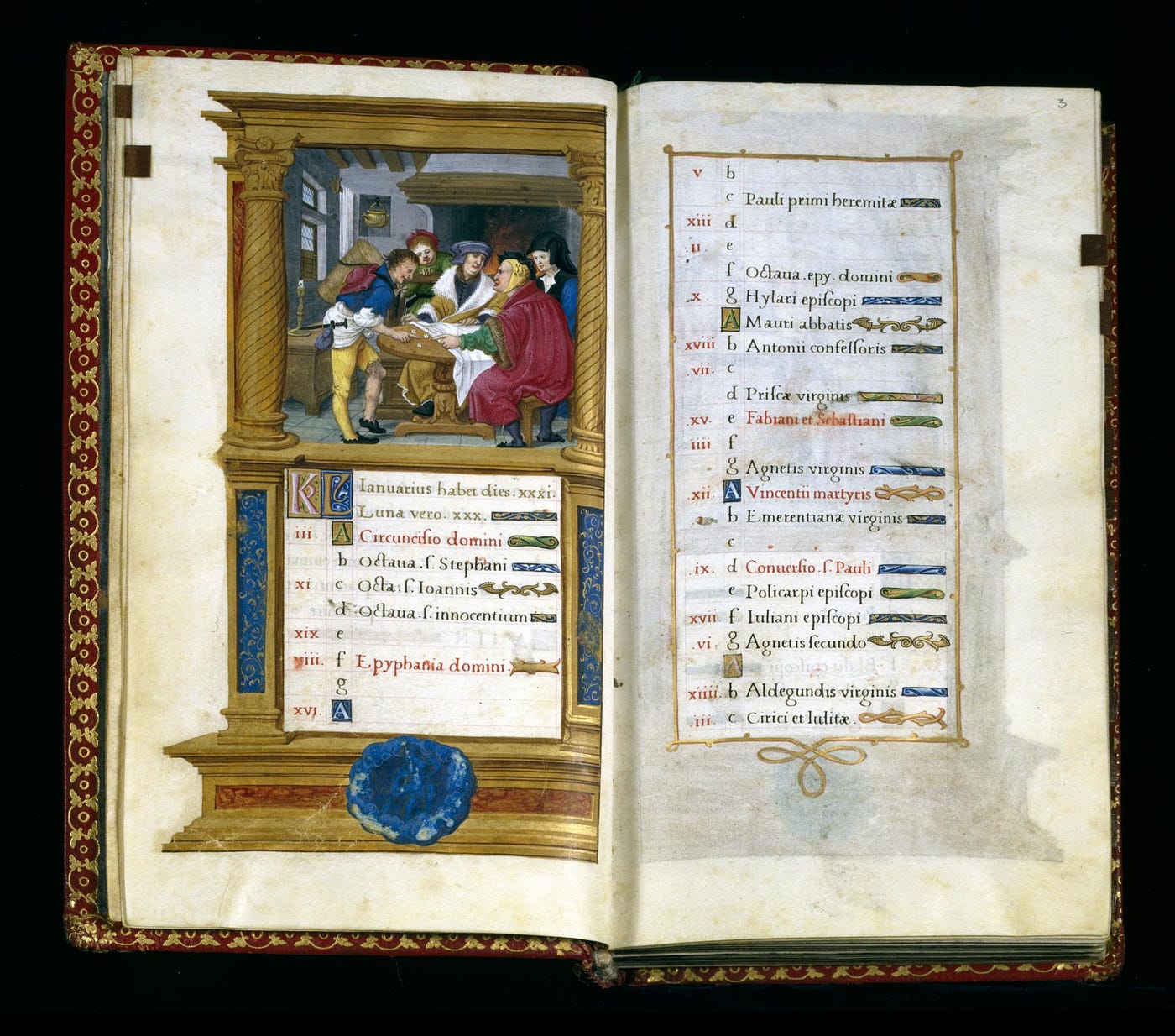The image captures two pages of an antique, vibrant, illuminated manuscript, likely dating back to the Middle Ages. The book, laying open on a black background, is bound with a maroon and gold embossed pattern along its edges. The left page features a divided layout: the upper half displays a colorful illustration bordered in red, showing five men in a dining room or main room, seated around a table. These men, dressed in a variety of vivid merchant attire, including reds, blues, whites, and yellows, are depicted examining a piece of white fabric. The central figure wears a blue hat and a white and brown coat, while others sport hats of different colors except for one, who remains bareheaded. The lower half of the left page includes markers on the edges and a section that appears to be a table of contents or inventory written in Latin. The right page is densely filled with similarly aligned Latin text, extending from Roman numerals III onwards, indicative of an extensive inventory list or continuation of the contents. The colors and inks have slightly transferred from one page to the other due to the book's age and the pressure of being closed.